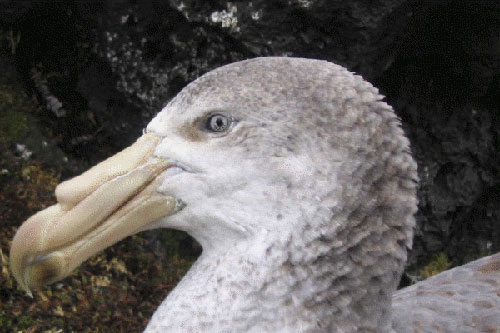The close-up photograph showcases the detailed head of an auk, a seabird known for its unique beak. The bird's head is turned to the left, yet its centered silver-gray eye gazes directly at the camera. The eye features a dark iris, adding to its striking appearance. The auk's beak is particularly noteworthy, displaying a light tan color with distinct channels that give it a layered, almost three-dimensional look—resembling an extra beak added onto it. The area around the beak and under the eye is predominantly white, contrasting with the short, gray feathers covering the rest of its head. The background consists of a rough, brown rock face, with a hint of green grass or shrubbery visible at the lower left of the image. Though the scene is sunlit, the overcast sky suggests a coastal or shoreline environment. The lower part of the bird's body is cropped out of the frame.